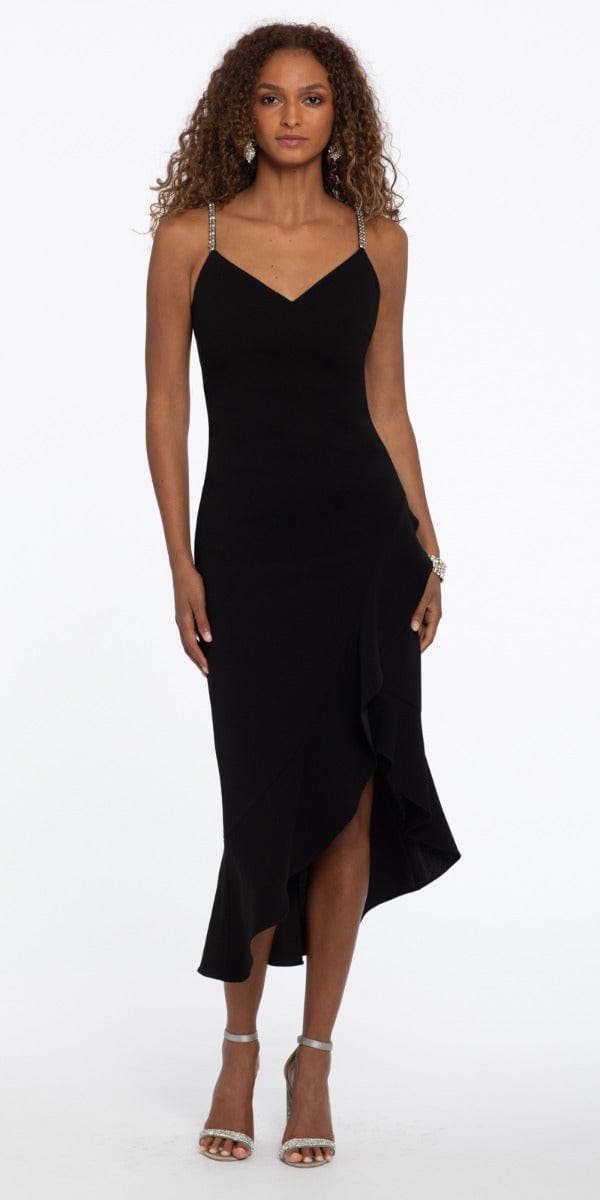The image features a tall, slender African-American woman in her mid to late 20s or early 30s, striking a poised and elegant modeling stance. She exudes beauty with her light brown skin and long, curly, brownish blonde hair that cascades down to her shoulders. She wears a strappy black evening gown with a V-neck, adorned with jeweled, clear rhinestone straps. The dress prominently features a high slit on the right side, showcasing her sophisticated style. Her accessories include a silver or diamond-like bracelet on her left wrist and matching silver drop earrings. She completes her look with minimal makeup and strappy, silver high-heeled sandals that feature ankle straps and rhinestone designs across the toes. The background is stark white, giving the appearance of a professional product photography session, possibly for an apparel website, with a faint shadow beneath her, adding depth to the otherwise pristine setting.